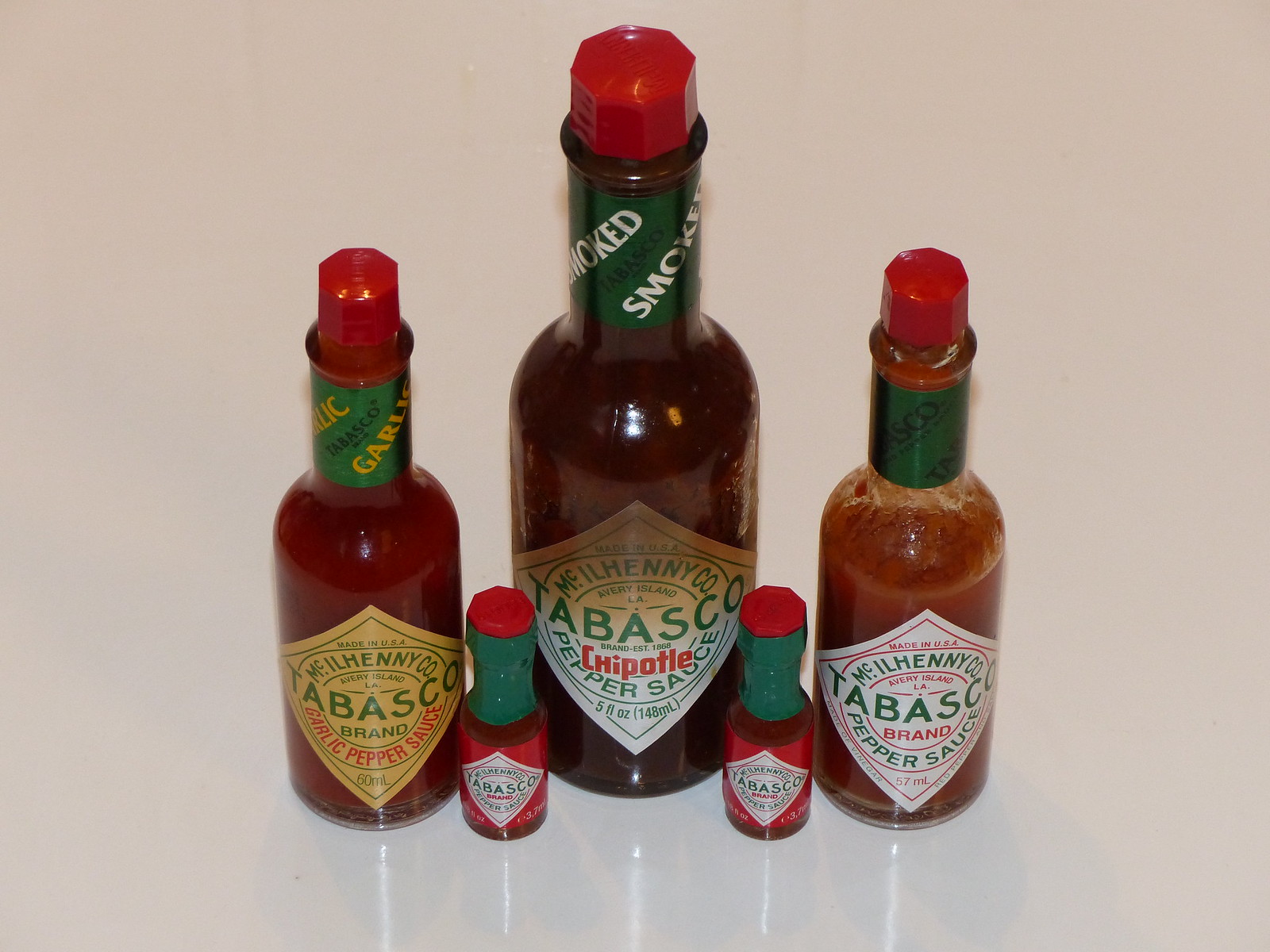The color photograph presents five bottles of Tabasco sauce arranged on a bright, glossy, white surface that reflects their presence. The tallest bottle, situated at the center, is a brown Tabasco Chipotle Pepper Sauce featuring a green strip around the neck with the word "smoked" printed diagonally in red and a vibrant red cap. Flanking this central bottle are two medium-sized bottles: the one on the left is unopened and has a yellow label denoting it as Tabasco Garlic Pepper Sauce, while the one on the right, with some sauce missing, displays a white label marking it as the standard Tabasco Pepper Sauce. Further flanking each medium bottle are two adorable, tiny mini bottles of standard Tabasco, each red in color with an unchanged green label and a red cap, sitting unopened. All bottles bear the iconic Tabasco branding with visible label text despite their differences in size and flavor variants. The arrangement on the gleaming surface, paired with subtle shadows, suggests a studio setting designed to highlight the distinctiveness of each bottle.